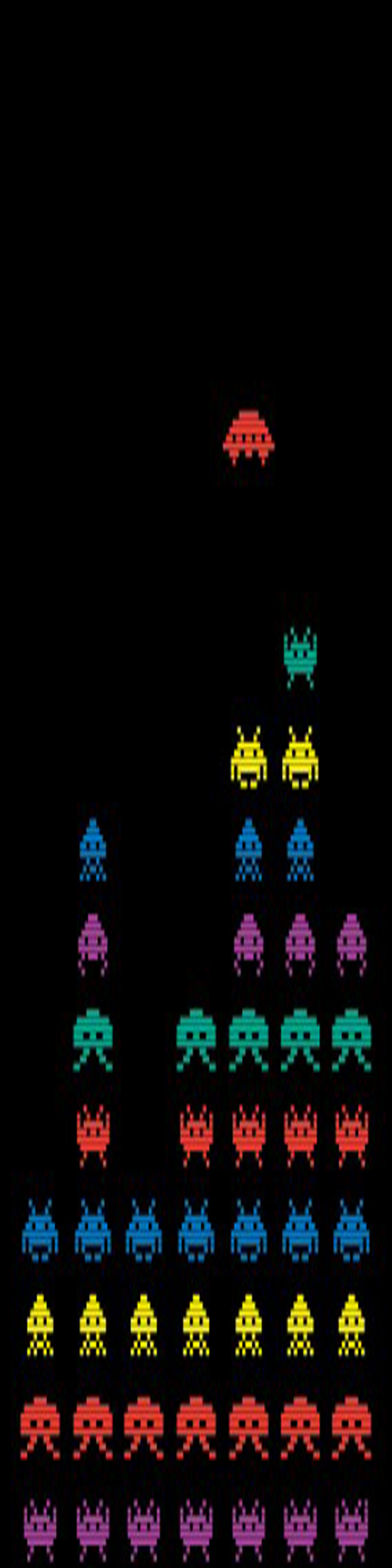The image is a tall, narrow, rectangular screenshot of a retro game reminiscent of Space Invaders or Galaga. The screenshot features a black background filled with colorful, pixelated alien invaders arranged in rows. At the top of the image, a red, UFO-shaped spaceship is visible, which appears to be in the process of shooting down at the rows of aliens below. The aliens are organized in a pattern, with the bottom row containing seven purple aliens, followed by a row with seven red aliens, then a row of seven yellow aliens, and above that, seven blue aliens. Higher rows begin to show gaps, indicating aliens have been shot out; for instance, one row has four red aliens on the right with a gap, another has four green aliens with a gap, and higher rows continue with similar irregularities. The aliens are in vibrant colors, including red, purple, blue, yellow, and green, set against the stark black backdrop. This detailed capture emphasizes the retro, pixelated aesthetic iconic to early video games.